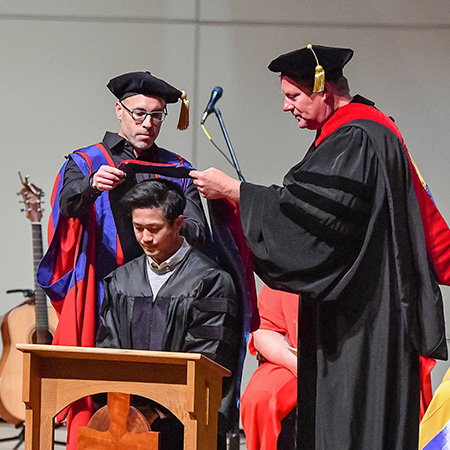In this detailed image of a graduation ceremony, a young Asian man with black hair is seated behind a small wooden podium draped in black robes. He is positioned at the bottom left of the image. Two men, both dressed in academic regalia, are standing behind and beside him. The man directly behind the seated individual wears a blue and red robe, black shirt, black cap, and glasses, and is holding a graduation cap over his head. The man to the right, dressed in black robes with a red collar and a black hat with a gold tassel, is also participating in the act, his face flushed red. To the far left of the scene, a guitar is visible, hinting at musical accompaniment, while a person in red clothing stands between the two men. The backdrop of the ceremony consists of a gray or white background, with additional people seated holding musical instruments and a microphone further emphasizing the formal and celebratory nature of the event.